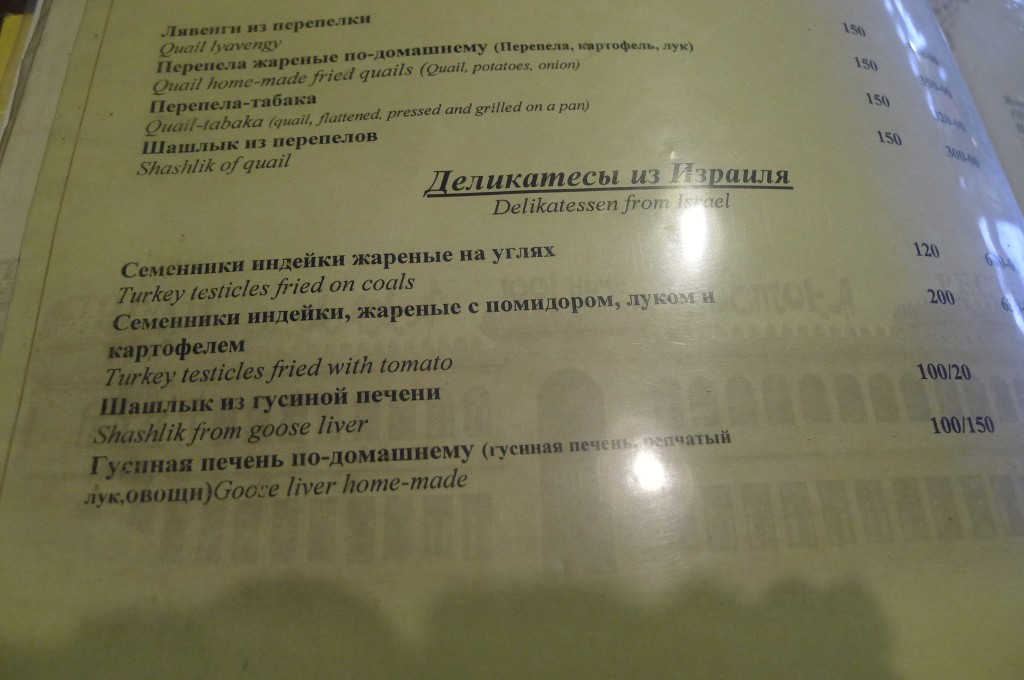In the photograph, a single page of a restaurant menu is displayed, capturing a blend of Hebrew and English text. At the center of the page, the words "Delicatessen from Israel" are prominently featured, accompanied by Hebrew script above it. The section of the menu visible in the image lists some notably exotic dishes. Among them, "Turkey Testicles Fries on Coals" is priced at $1.20. Another item mentioned is "Turkey Testicles Fried with Tomato." Additionally, the menu offers "Shashlik from Goose Liver," described as homemade goose liver. Further down, you can find "Shashlik of Quail" and "Quail Taboca." The variety of items suggests a unique culinary experience emphasizing traditional and adventurous delicacies available at this Israeli restaurant.